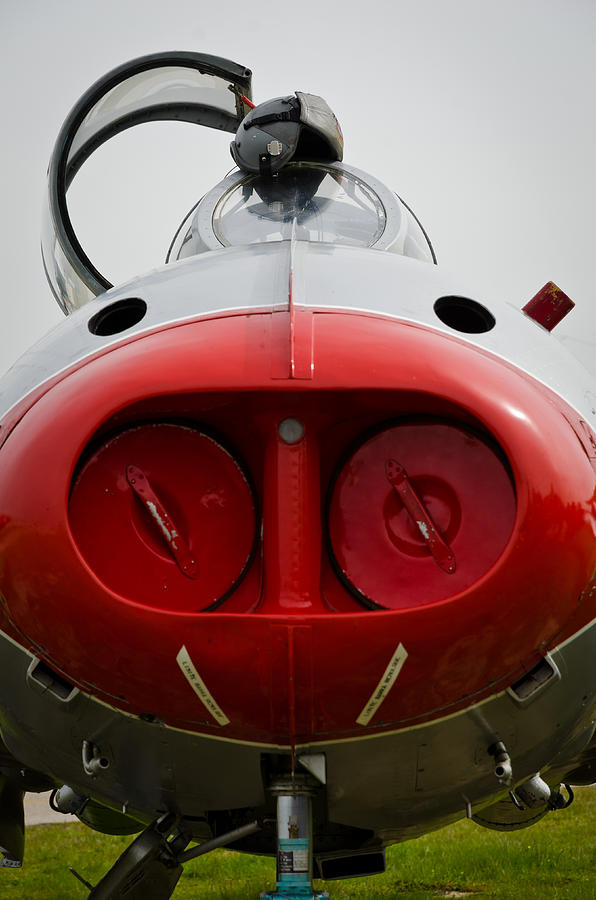This image is a detailed, color photograph in portrait orientation, showcasing a bizarre and highly modified aircraft or spacecraft reminiscent of a futuristic drone. The image captures a close-up view of the vehicle's front, focusing on several notable features. 

The nose of the vehicle is painted a striking red and is conical in shape. Central to this nose section is an opening, revealing the interior which houses two large, red canister-like lids, complete with handles, flanked by vertical steel components. These lids appear as if they can be unscrewed, adding curiosity to their functionality in such a vehicle. Surrounding this central opening are two black elliptical shapes positioned symmetrically on either side, adding to the mechanical aesthetic.

A bubble-shaped dome made of clear, elliptical glass panels sits atop the aircraft, likely serving as the cockpit for one or two occupants. The glass structure extends with additional side panels and is perched within a gray curved body. At the very top of this dome, there is something resembling a black helmet, adding an element of intrigue and possibly hinting at an automated or robotic feature.

To the left of the dome sits an opened convex hatch door, supported by a red hinge, which is bordered by black plastic and filled with clear glass. Below the nose section, some landing gear is visible towards the bottom left, complementing the photo's earth-bound setting with green grass and a cloudy gray sky framing the scene.

The overall design and features of this vehicle, merging elements of military aircraft and space-faring technology, present a perplexing yet captivating visual that remains open to interpretation.